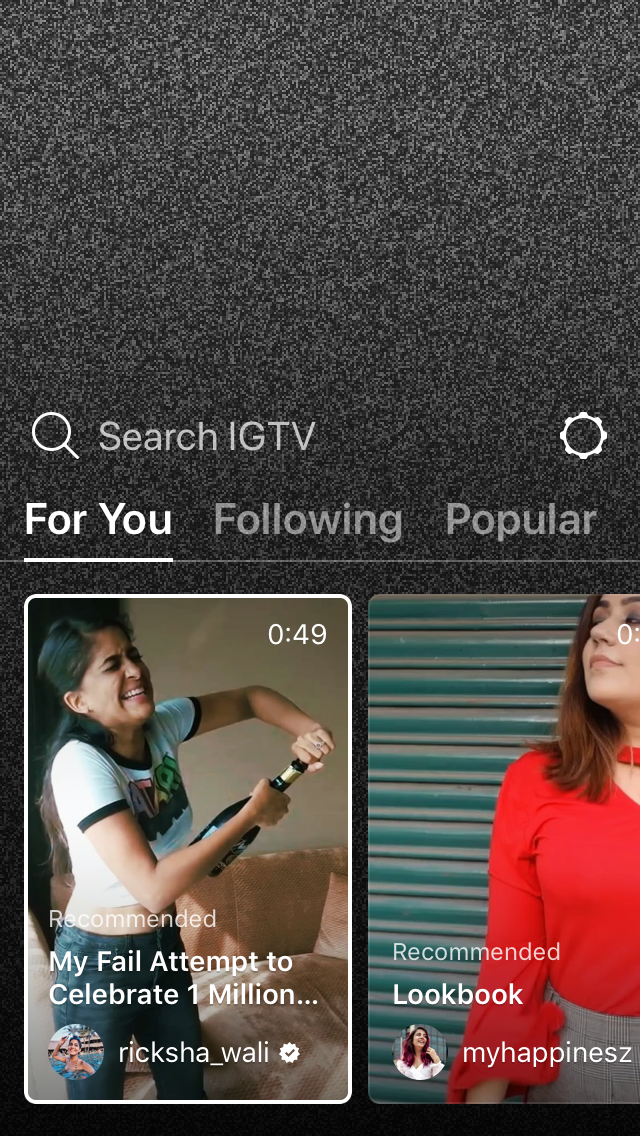A black and white, grainy image captured from a phone screen, predominantly gray and somewhat indistinct towards the top. In the clearer lower section, you see a white magnifying glass icon next to the text "search IGTV," followed by a clickable white gear icon, suggesting settings access. Below this row are three tabs labeled "For You," "Following," and "Popular." The "For You" tab is highlighted in white, indicating it's selected, while the other two tabs are in gray.

The first prominent visual element shows a girl struggling to open a wine bottle, her face contorted in a grimace. The video is 49 seconds long, captioned "recommended my fail attempt to celebrate 1 million." Adjacent to this video is another labeled "recommended look book, my happiness," featuring a girl in a red shirt.